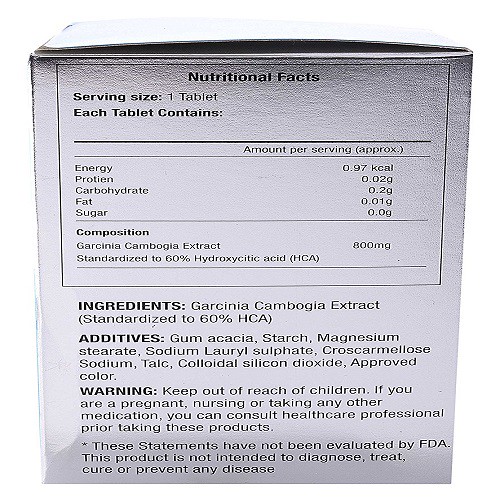The image depicts a segment of a shiny silver box, likely a nutritional supplement packaging for tablets. The side of the box showcases detailed nutritional facts in black print, with "Nutritional Facts" prominently displayed at the top. Below this, a table outlines the contents per serving size of one tablet, listing the amount of energy (0.97 kcal), protein, carbohydrates, fat, and sugar. The key ingredient noted is Garcinia Cambogia extract, standardized to 60% hydroxycitric acid (HCA), with additional additives specified. Important information is emphasized in bold capital letters, including ingredients, additives, and a product warning about keeping the supplement out of reach of children and precautions for pregnant or nursing women. A disclaimer at the bottom states that the product has not been evaluated by the FDA. The photo captures the slight reflective quality of the box, hinting at its handled state or the effect of an overhead light source.